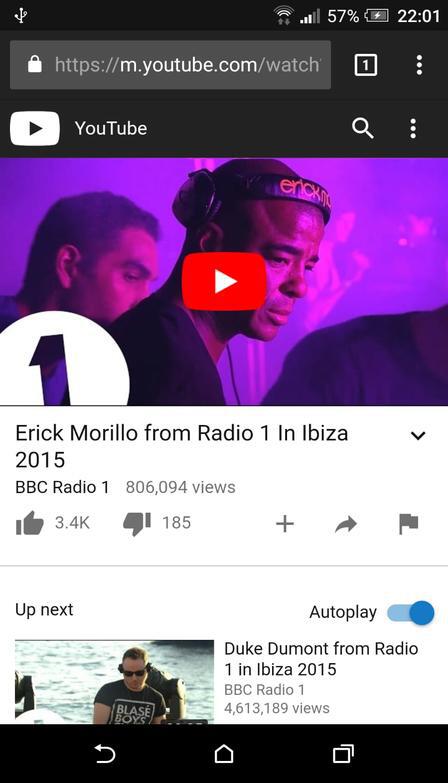Screenshot of a YouTube webpage displaying a paused video. The video interface reveals a battery life of 57% and a timestamp of 22:01 in the top right corner, indicating the current time. Only one tab is open, showing a "1" next to the YouTube logo, indicating this is the only active tab.

The YouTube logo here is in reverse color scheme; rather than the usual black play button on a red background, it is depicted in white with the word "YouTube" in white. Adjacent to the magnifying glass search icon, there are three vertical dots—representing additional options.

The paused video features a DJ, identified as Eric Morillo at Radio One IBIZA 2015. Eric, a Black man, is wearing headphones and a black shirt, standing behind a DJ set with another person visible in the background, suggesting a club setting. The video has a red play button at the center. Video statistics show 3,400 likes and 185 dislikes, along with options to add to playlists, share, and report the video.

Below the paused video, the "Up Next" section displays a thumbnail of another DJ, a white man wearing sunglasses and a black shirt labeled "Blase Boys," seemingly performing near a body of water. The video, titled "Duke Dumont from Radio One," boasts over 4 million views.

At the bottom of the screen, a black navigation bar features buttons for going back, a home button, and a button to view multiple tabs.